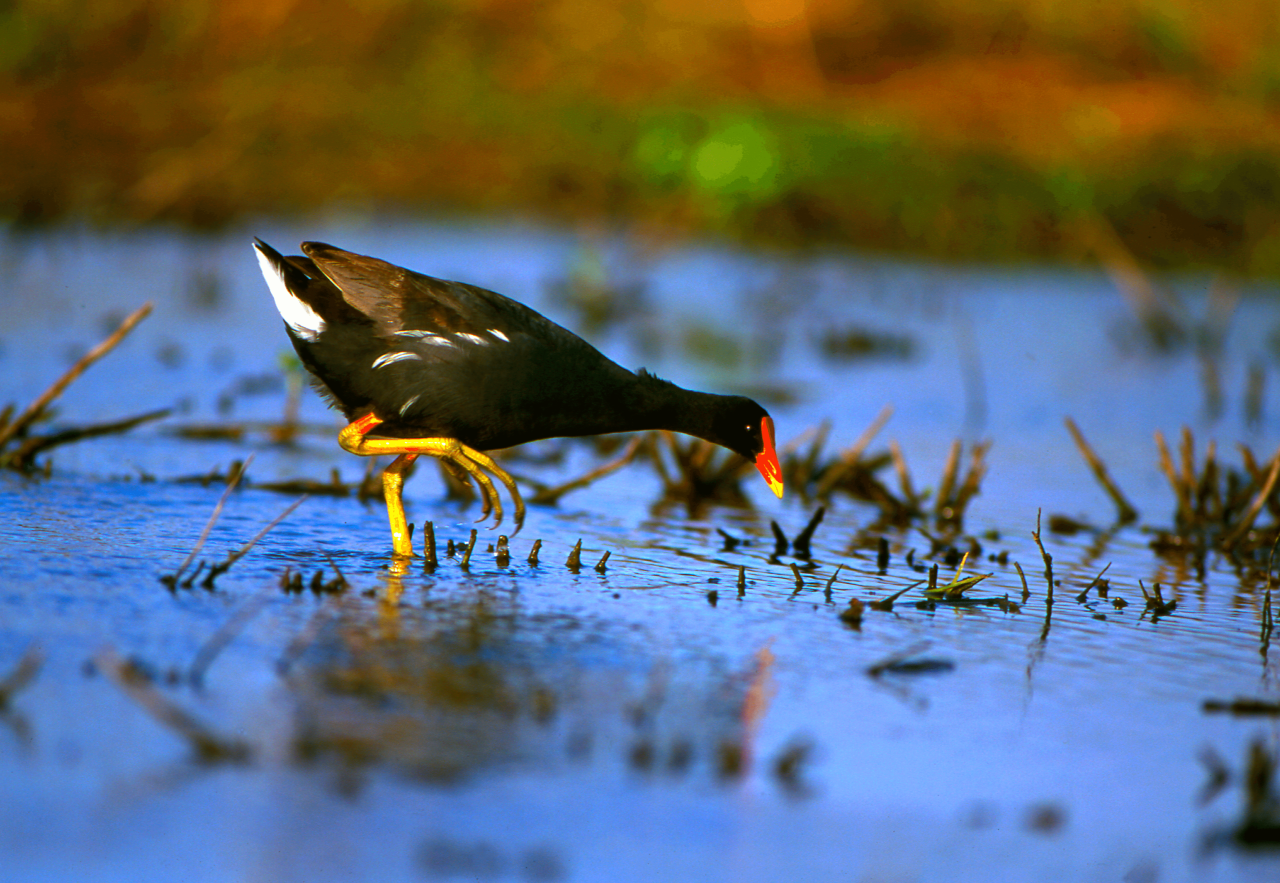The image captures a striking scene of a black bird with vivid yellow legs, large yellow claws, and an orange beak with a yellow extension, cautiously navigating through a shallow, light blue, reflective puddle. The bird, which features white accents near its wings and on its backside, is poised with one leg in the water and the other lifted parallel, as it pecks intently, likely in search of food. The water is interspersed with little brown sticks, roots, and plant stems, adding to the natural ambiance of the habitat. The background, a soft blur of brownish-orange and green hues, suggests a lush, vegetative environment, emphasizing the bird's focus and the serene, yet lively, setting.